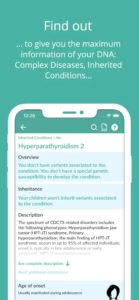In the intentionally blurred image, the text in the top middle reads "Find out..." suggesting a continuation of information. Below, in a smaller font, it says, "to give you the maximum information about your DNA, complex diseases, inherited conditions..." Following this ambiguous teaser, the central part of the image features a photo of a smartphone displaying a website. The smartphone's border is white, and its interface appears realistic, perhaps suggesting a visual representation of a real device.

At the top of the phone's screen, a rectangular bar crosses the width with a small circle on it, possibly simulating a camera lens. The status bar at the right corner includes a fully charged battery icon and a full Wi-Fi signal icon. The left corner shows the time as 12:28. Adjacent to these indicators are three icons at the top middle-right: a magnifying glass (search), a piece of paper (possibly a document or notes), and a white circle containing a black question mark (help or information).

Central to the phone's display is the term "hyperparalysis 2," flanked by two boxes labeled "Overview" and "Inheritance," hinting at sections of content related to the term. Further down, the word "Description" is visible, followed by detailed text that is largely unreadable due to the image's blur. The entire setup seems to be a digital interface designed to provide detailed genetic information and related medical insights.